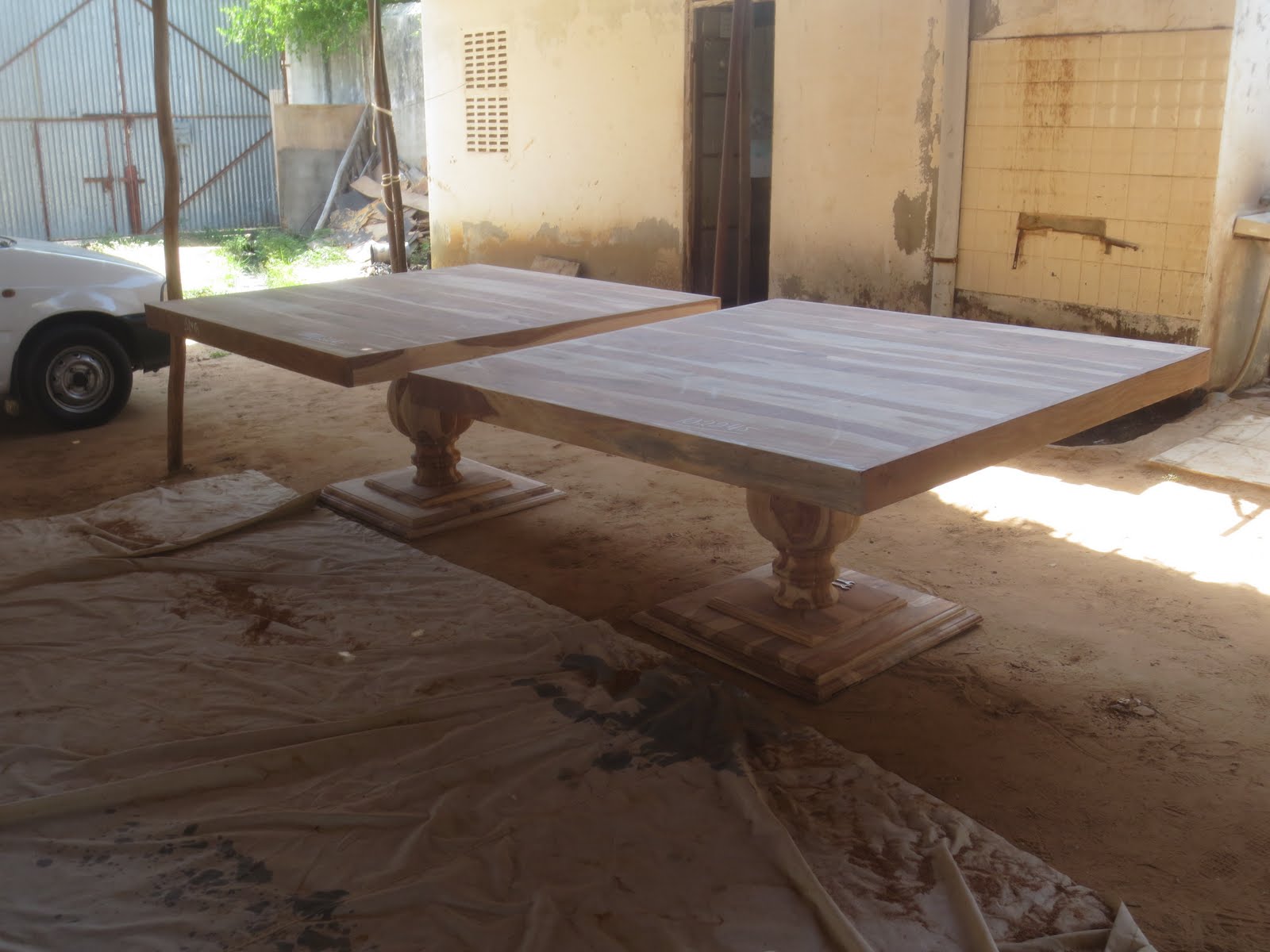In this outdoor image, likely taken during the day in a tropical or warm season, we see a detailed workspace set under a work tent. On the far left, there's an old metal building partially covered in green grass and shrubs. Nearby, part of a white vehicle is visible. The tent structure is letting some sunlight filter through, illuminating two large, square, wooden tables with intricate, statue-like bases, possibly awaiting staining. Between the tables and the tent, there's a white sheet sprinkled with wood shavings. The ground beneath the workspace is dirt-covered with a tarp laid out to protect it. In the background, a tan, clay-like building is noticeable, flanked by an industrial-type structure made of metal sheets. The scene is lively with elements of woodworking in progress amidst a mix of natural and artificial surroundings.